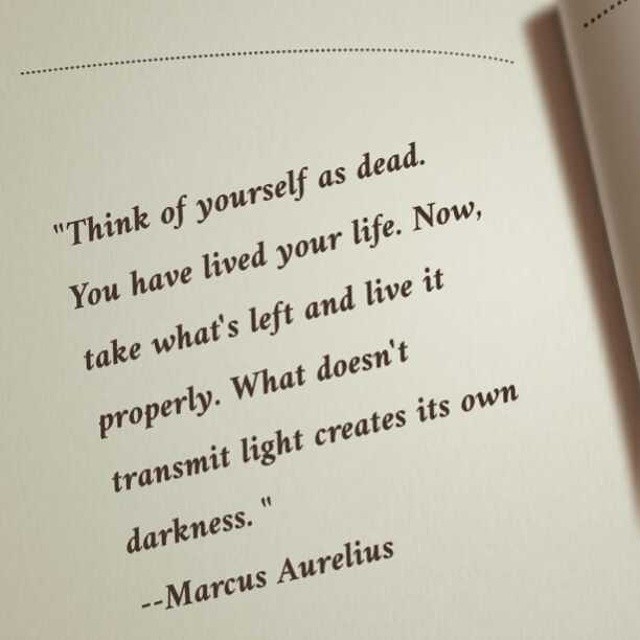The image is a detailed excerpt from a book, showcasing a powerful quote by Marcus Aurelius. The page, positioned on the left side of an open book, features a light green background with black text. Across the top of the page, there's a line of small black dots. The primary focus is the impactful quote, "Think of yourself as dead. You have lived your life. Now take what's left and live it properly. What doesn't transmit light creates its own darkness." attributed to Marcus Aurelius. The quote is written in a brownish-gray font. In the upper right part of the image, part of the adjacent page is visible, showing a similar dotted line pattern and casting a shadow onto the main page. Overall, the image has a minimalist, yet profound and inspiring presentation.